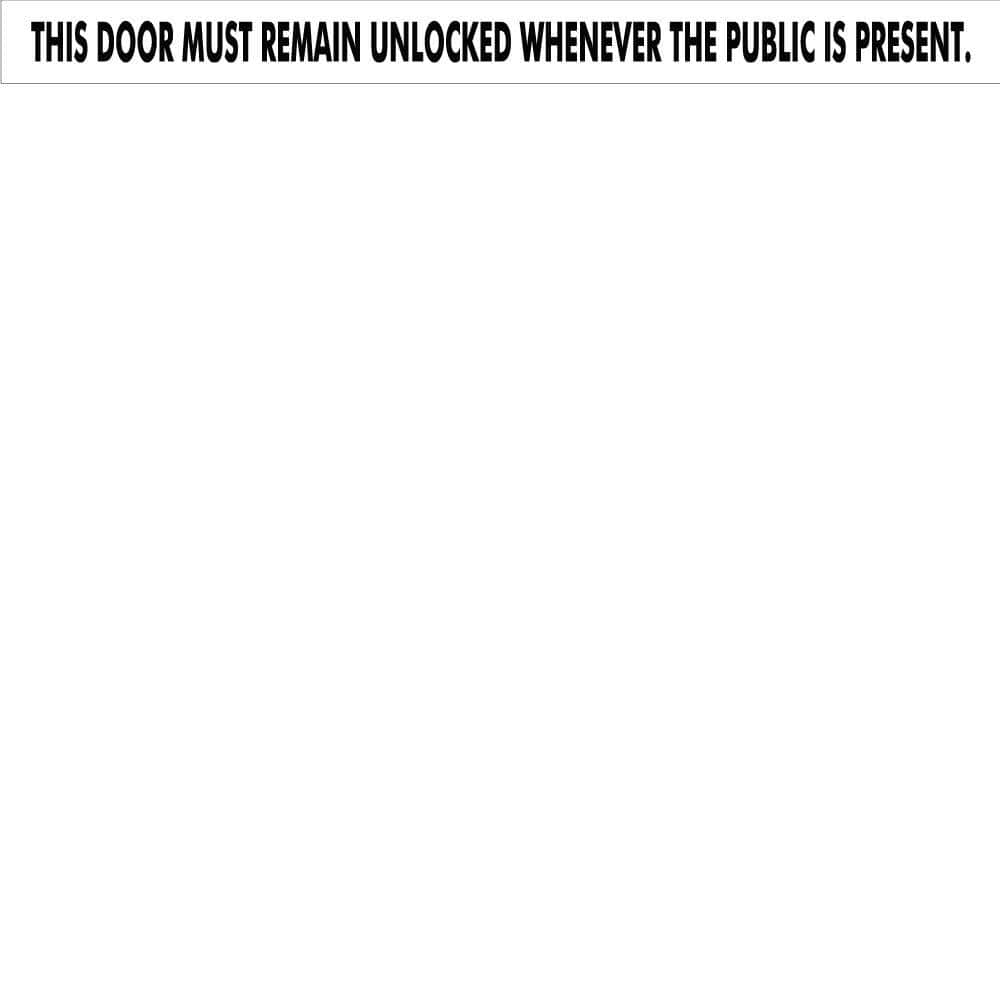This image is a horizontally-oriented, very thin rectangle. The image is bordered on the left, top, and bottom sides with a fine black line, leaving the right side open without a border. The background of the image is transparent, revealing the white background of the computer screen behind it. Centered in the image is a message written in bold, black, uppercase letters. The text reads, "THIS DOOR MUST REMAIN UNLOCKED WHENEVER THE PUBLIC IS PRESENT," and is followed by a period. The font is thick with the letters closely spaced, giving a compact appearance.